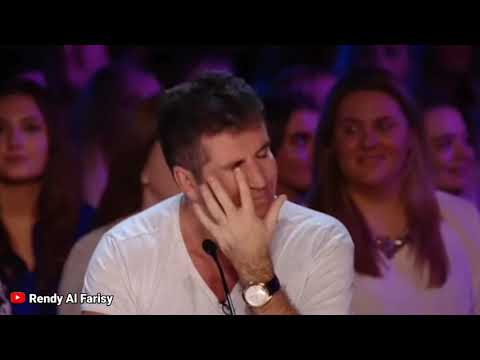This is an image of Simon Cowell, seated and wearing his signature white V-neck T-shirt, captured in what appears to be a screenshot from a TV show, potentially 'America's Got Talent' or 'American Idol'. He is seen with his right hand touching his face, specifically his right eye, and his eyes are closed, giving an impression of a shy smile or amusement. Cowell is wearing a black wristwatch with a white round face on his left wrist. In front of him, there's a small microphone indicating he might be involved in a judging or commentary role. The background is a blurred audience, who appear to be surprised and are looking in various directions. A conspicuous element is the YouTube logo in the bottom left corner, accompanied by text that reads "Rendy Alf Faresi" or a similar name, suggesting this is a still from a video posted on YouTube. The image is framed by black headers and footers, typical of a video playback screen.